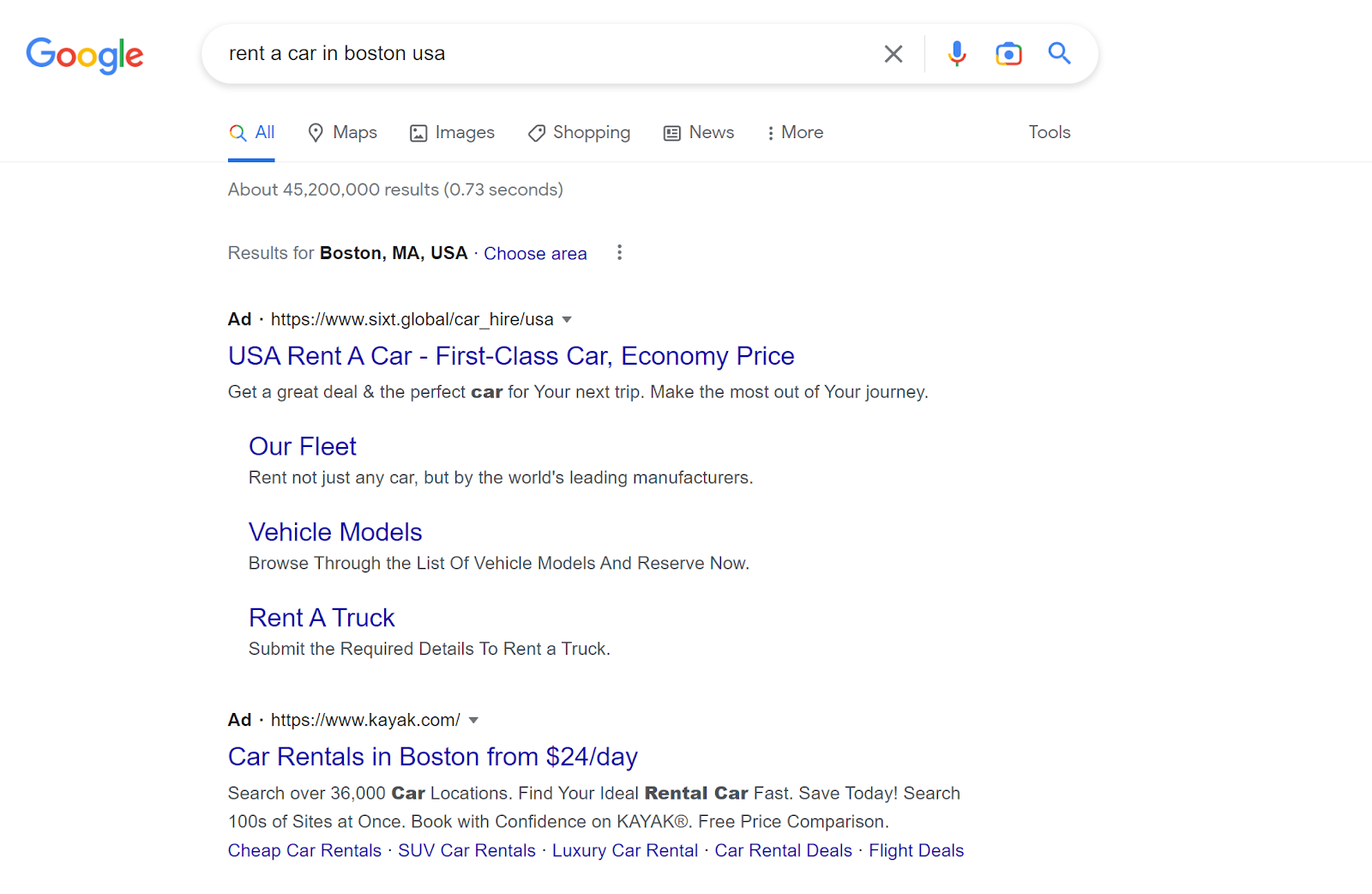This image displays a Google search results page. At the top left, the iconic multicolored Google logo is prominently visible. Directly to its right lies the white search bar containing the user's query, "rent a car in Boston, USA." Adjacent to the search bar, the familiar symbols for voice input (microphone), image search (camera), and text search (blue magnifying glass) are neatly aligned.

Below the search bar, the menu tabs 'All,' 'Maps,' 'Images,' 'Shopping,' 'News,' and 'More' offer options to refine the search, with the 'Tools' button situated on the far right for additional settings. The search has yielded approximately 45,200,000 results in a swift 0.73 seconds, as indicated just beneath these tabs. 

The results section starts with an ad from Sixt, highlighted at the top, featuring options for 'USA rent a car,' 'First class car,' 'Economy price,' and quick-access tabs for 'Our Fleet,' 'Vehicle Models,' and 'Rent a Truck.' Directly following this ad is another sponsored link from Kayak, advertising car rentals in Boston starting from $24 a day.